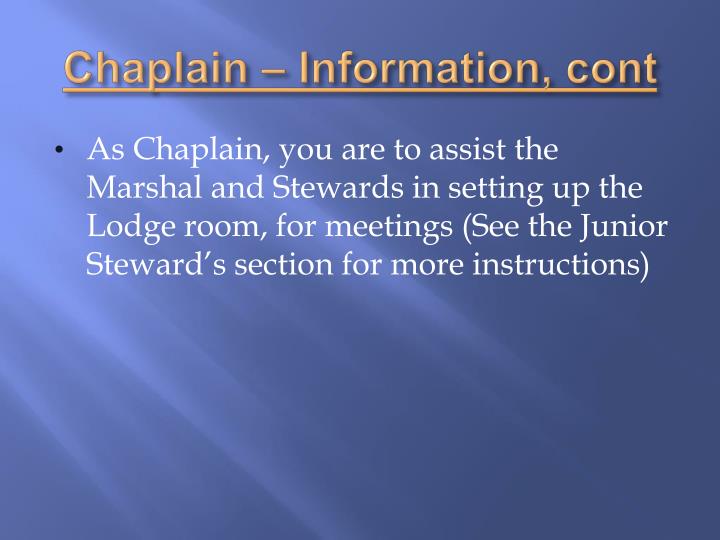The image depicts a PowerPoint slide with a medium blue background adorned with light blue streaks emanating from the upper left corner. Centered at the top is a title in yellow-gold text with an underline of the same color. The title reads: "Chaplain - Information, CONT," presumably short for "continued." Below the title, there is one black bullet point followed by four lines of white text. The text reads: "As chaplain, you are to assist the marshal and stewards in setting up the Lodge room for meetings. (See the junior steward section for more instructions.)" The slide's simple composition includes the yellow-gold title and a single bullet point about chaplain duties, prominently displayed in white text.